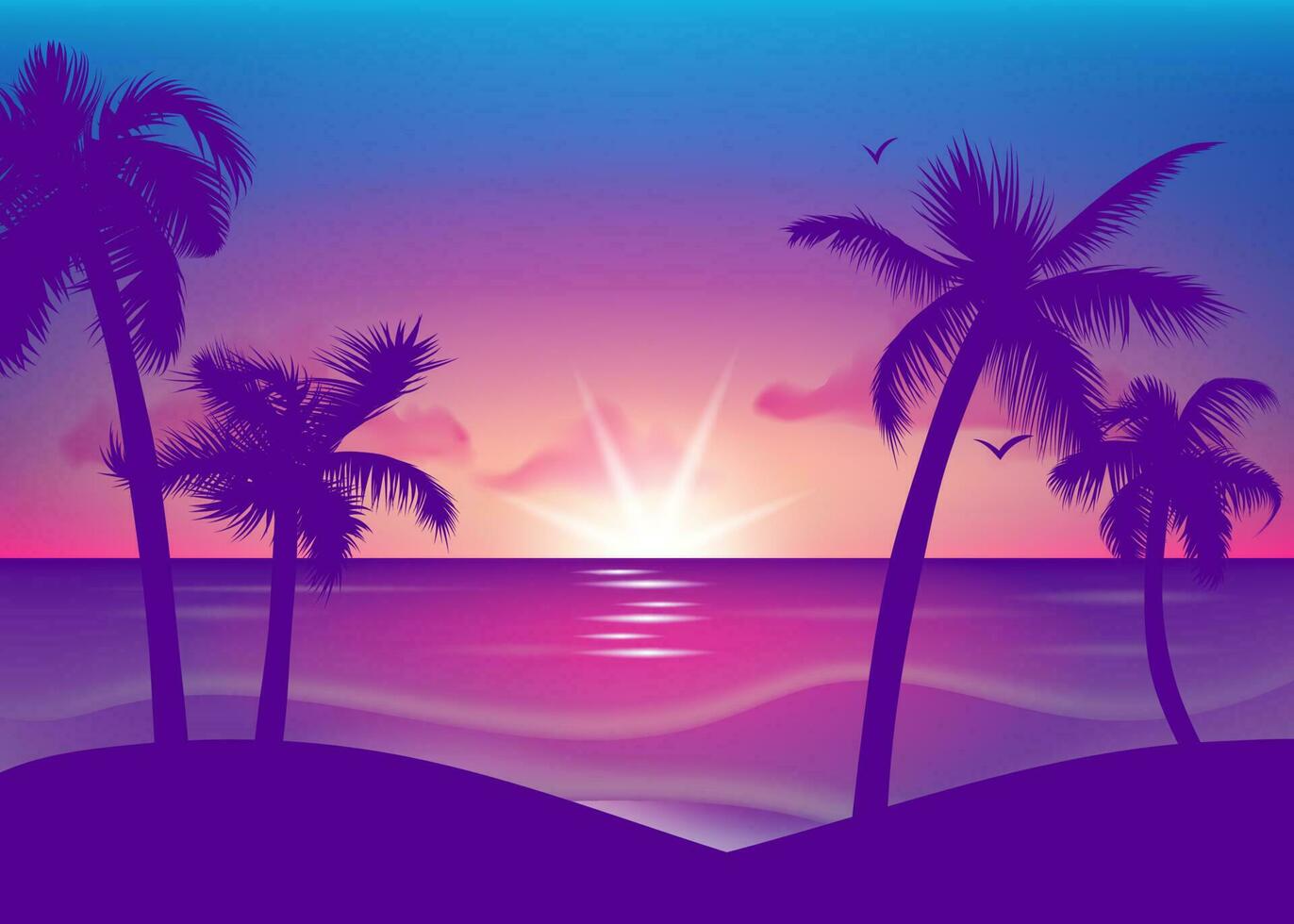This stylized digital depiction of a tropical beach scene captures an 80s Miami Vice vibe with its vibrant, exaggerated colors and silhouettes. At the forefront are two deep purple mounds, each supporting a pair of silhouetted palm trees. The left pair leans gently to the left, while the right pair curves slightly to the right, creating a mirrored effect. In the backdrop, a pink sea with light gray waves stretches across the frame, dotted with white bursts of light. The sun, half-submerged on the horizon, radiates four bright rays, setting the sky ablaze in gradients of orange and pink that transition into a bright electric blue at the top. Two stylized checkmark-shaped birds, also in deep purple, soar near the right set of palm trees—one above the left-center tree and one below it. The scene is framed without any text or identifying marks, emphasizing its strong visual style.